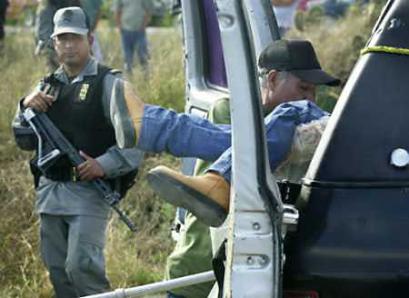The image depicts a tense scene, possibly indicative of a crime scene or a war zone. Central to the scene, there are two patrol officers situated beside a white van with its side doors open. The officer to the left is wearing a light gray baseball cap, a black vest with a badge on his left chest, a gray shirt, and gray pants. He is holding a sizable assault rifle pointed towards the ground. The second officer, positioned closer to the van, is wearing a black baseball cap. He is in the process of lifting a person out from the rear side of the van, whose legs clad in blue jeans and tan boots with black soles are visible.

The setting is an open, grassy field, characterized by tall grass. In the background, a few more individuals are present, their heads cropped out of the frame, emphasizing their distance and the vastness of the field. The scene is dramatic and intense, with the officers seemingly focused on a significant task at hand amidst the uncertainty painted by the distant figures.